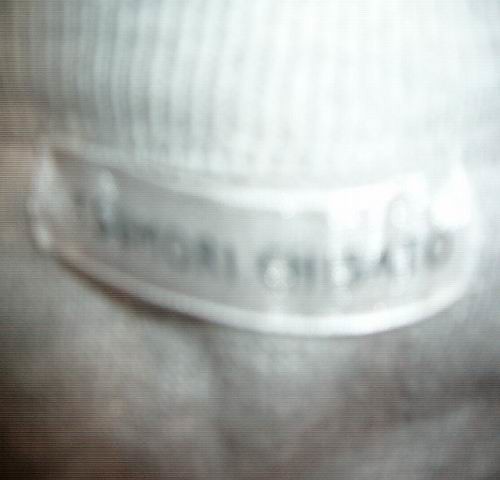The image depicts a piece of cloth featuring a partially visible label. The label appears slightly bent, making it challenging to read. However, parts of the text can be discerned, with "M-O-R-I" visible on one side, followed by a space, and then "C-H" and possibly "I-S." The label itself is characterized by black text set against a grey background, bordered by a light grey trim. The label seems to be affixed to a garment, which might be a hat given the visible features. The garment below the label is greyish in color, consistent with the fabric's texture. The upper section of the garment presents a different design yet is still grey and fabric-like in appearance.